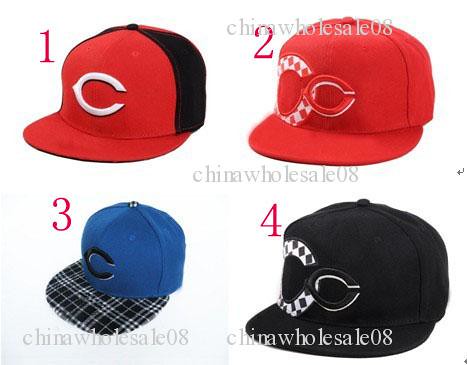The image showcases four distinct styles of baseball caps displayed in a floating grid formation against a white background. Each cap is marked with a bold red number in a serif font, denoting their positions: the top left is 1, the top right is 2, the bottom left is 3, and the bottom right is 4. A gray watermark reading "China Wholesale 08" is scattered across the image, visible in the center, bottom left, bottom right, and top right.

In the top left corner, the first cap is predominantly red with a white embroidered 'C'. It features black panels on the side sections and the button on top, creating a striking contrast. The brim matches the red color of the cap. The second cap, located at the top right, is entirely red, inclusive of a red 'C' with white shadowing for depth, and a larger checkerboard 'C' in white and red on the left side.

The bottom left quadrant holds the third cap, a navy blue design with a black embroidered 'C' outlined in white. This cap's brim stands out with a black and white tartan plaid pattern, providing a unique visual texture. Finally, the bottom right cap is black with a black 'C' that features a white drop shadow, complemented by a larger checkerboard-patterned 'C' filled with a black and white design to the left.

Overall, the detailed descriptions of the caps, their colors, lettering, and patterns, along with the positioning and watermark placements, capture the varied designs and structured layout of this product image.